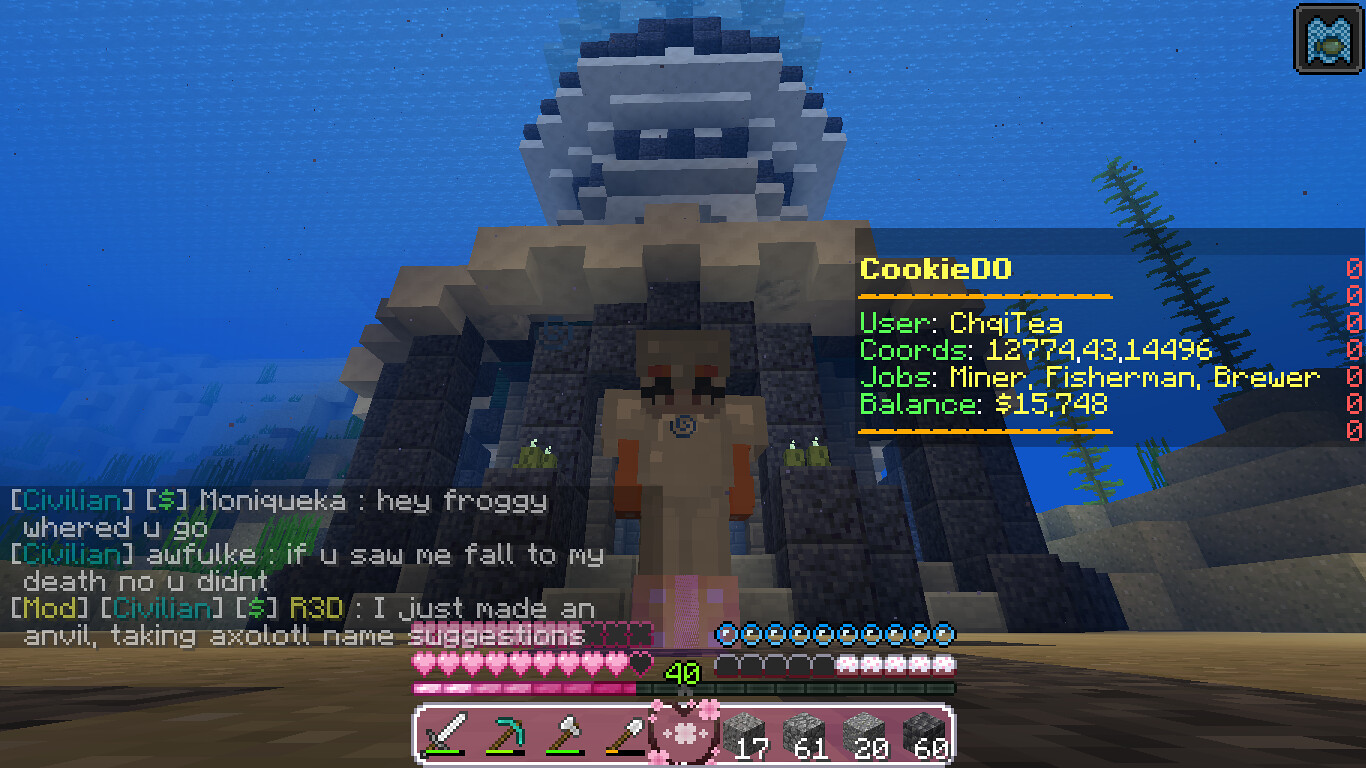The image appears to be a screenshot from an old, pixelated video game with low resolution. The scene depicts a large, blocky, stone-like temple or monument reaching up towards a sky composed of square blue blocks, creating a unique Lego-like effect. The monument consists of various layers in shades of gray and beige, with the upper section exhibiting gray and black hues. It features a beige block figure that somewhat resembles a face with dog-like features, including orange arms and pink block-like feet. In the foreground, the ground is made up of beige and brown blocks, and the right side of the image shows some stick-figure-like trees and stairs leading upwards. On the left side of the screen towards the bottom, there is a chat box with white letters. Various scores in yellow and green letters are displayed on the right side of the screen, and control panels featuring emojis and information about the player’s coordinates, jobs, and balance are positioned at the bottom center and right of the screen, respectively.